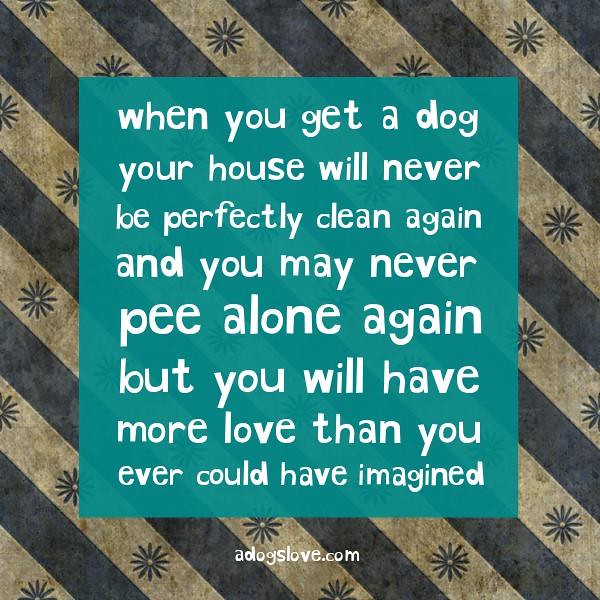The image features a diagonally striped background with alternating dark brown and lighter brown stripes, decorated with darker brown flower patterns on the lighter brown stripes. Superimposed on this background is a teal rectangle containing white text that reads, "when you get a dog, your house will never be perfectly clean again, and you may never pee alone again, but you will have more love than you ever could have imagined." At the bottom center of the image, on the striped background, is the website name "adogslove.com" written in lowercase white text without punctuation. There are no people or additional images present in the picture.